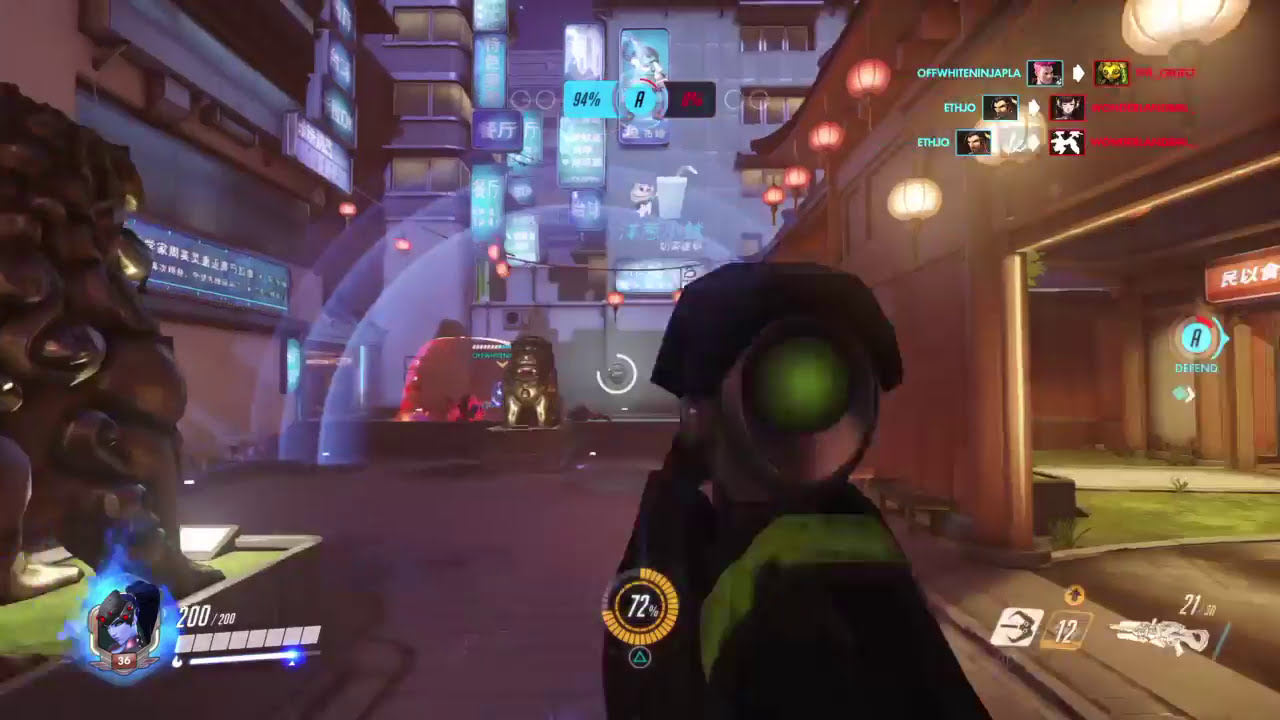The image is a highly detailed screenshot from a futuristic first-person shooter video game set in a vibrant, neon-lit cityscape. Dominating the foreground is a large rifle with a night vision-like green lens scope, perfectly centered along with the crosshairs for aiming. The background reveals an intricate alleyway featuring various illuminated structures, including a statue of a lion on the left and a temple adorned with Chinese lanterns on the right. The scene is bustling with signs in Chinese characters and illuminated by a myriad of colors: brown, green, blue, purple, white, black, orange, yellow, tan, and red.

The heads-up display (HUD) is packed with information. In the bottom left, there is a health bar icon next to a profile picture of a purple female character marked with the number 36. The bottom center features a power-up percentage display at 72%, while the bottom right shows the player's inventory, including a futuristic gun icon. At the top of the screen, a blue section indicates a score of 94%, accompanied by a smaller blue circle with an "A" inside it and a black section displaying 8%. The upper right corner reveals a kill feed with blue and red text signifying different teams, suggesting that this is a multiplayer game. Additionally, markers on this part of the screen indicate the locations of other players. This detailed setting and the rich HUD elements make the image an engrossing snapshot of the game's dynamic and immersive environment.